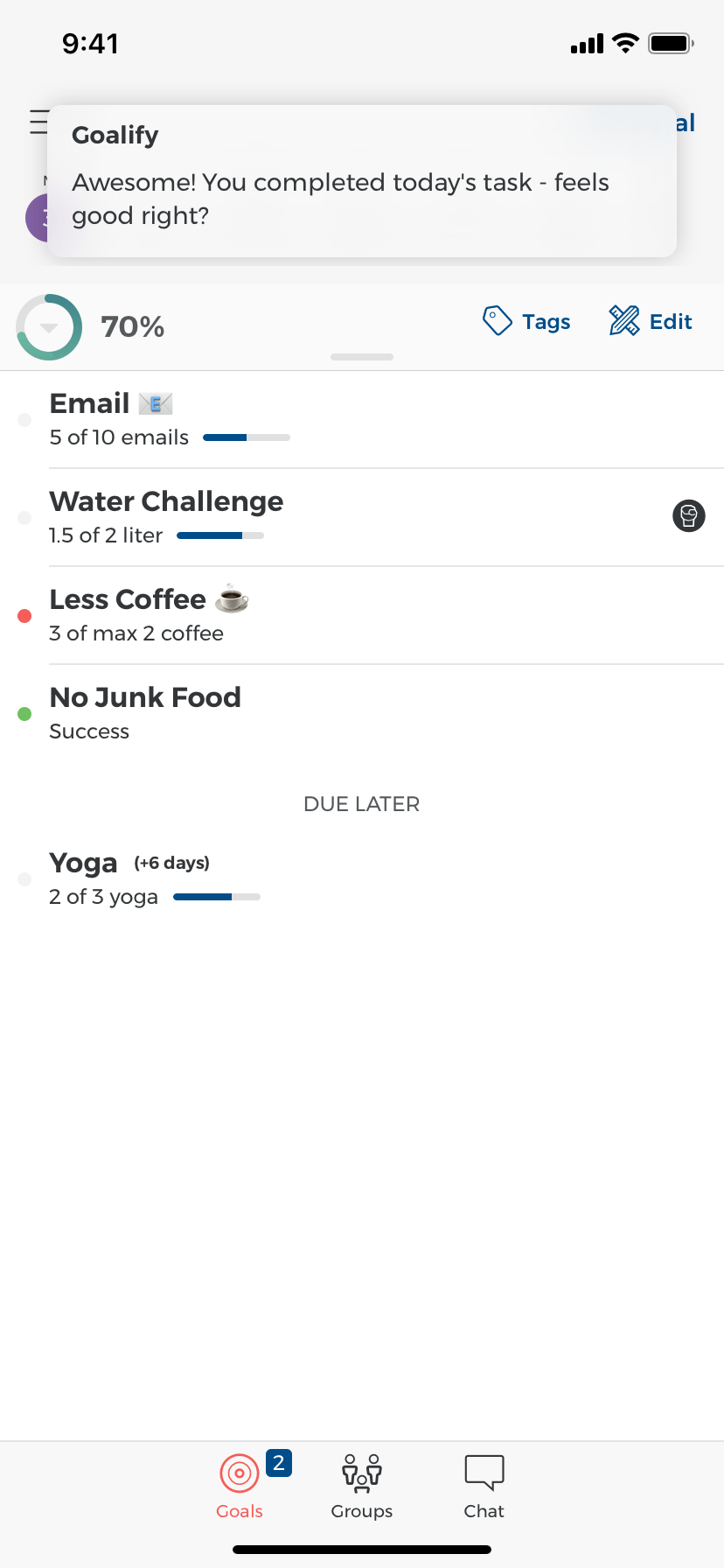Detailed Caption: 

The image is a screen capture of a smartphone at 9:41 am, with a nearly depleted battery. At the top of the screen, a notification from the Goalify app reads, "Awesome! You completed today's task. Feels good, right?" Below the notification, the screen displays various metrics and tasks associated with daily goals. A progress bar shows 70% completion, with sections titled "Tags" and "Edit."

The email section indicates that 5 out of 10 emails have been addressed. A water intake challenge shows that 1.5 out of 2 liters of water have been consumed. There is an urgent warning highlighted in orange for excessive coffee consumption, showing 3 of a max allowed 2 coffees. Success is noted in green for avoiding junk food, with a subsequent task labeled "Do later" referring to yoga. Progress on yoga is logged as 2 out of 3 sessions completed within the past six days. The interface suggests an ongoing effort to enhance daily performance and health.